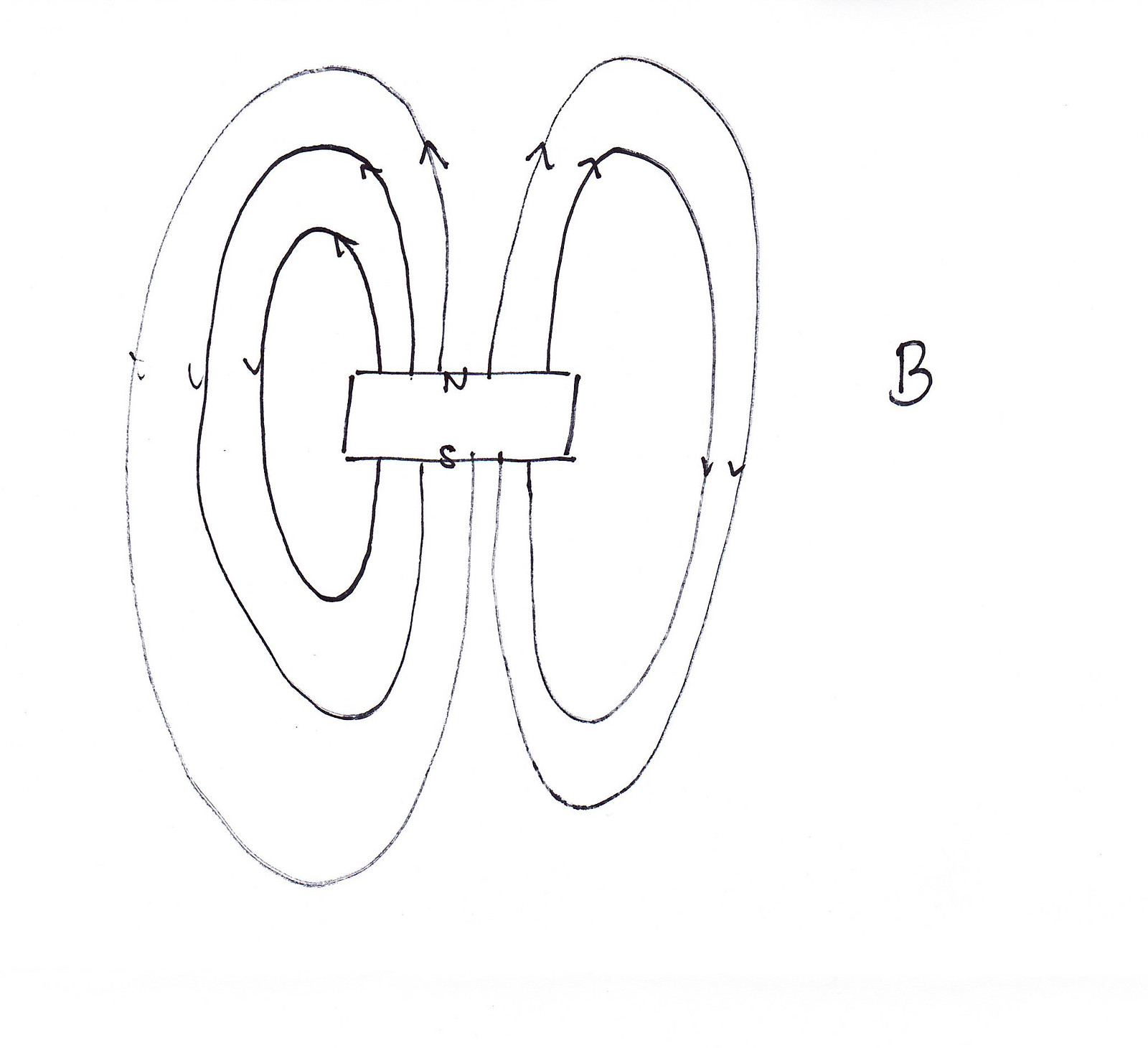This photograph captures a hand-drawn diagram on a white sheet of paper, executed with a fine-tip black marker. The diagram features prominent geometric shapes, primarily circles and a rectangle, which are likely part of a mathematical or scientific illustration.

On the right side of the paper, an uppercase letter "B" is noticeable. The diagram is mainly divided into two parts by a central rectangle. On the left, there are three concentric circles: a large outer circle, a medium circle nested within it, and a smaller circle at the center. These circles have arrows pointing to the left, indicating a counterclockwise direction.

Conversely, on the right side, there are two circles: a larger outer circle encompassing a medium-sized inner circle. These circles feature arrows pointing to the right, signifying a clockwise direction.

The central rectangle connects the two sets of circles. At the top of the rectangle, the letter "N" is marked, while at the bottom, the letter "S" is present. The diagram’s layout suggests it represents some form of rotational system or magnetic field, given the directional arrows and labeled letters.

Overall, this detailed and well-organized diagram lacks any additional identifying marks or context, implying it might be an instructional tool for a math or science class, focusing on the calculation and understanding of the illustrated elements.